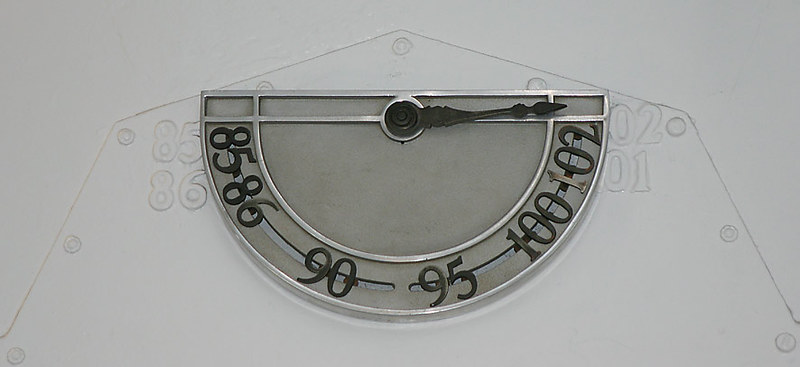This detailed image showcases a hybrid of photographic and penciled elements which combine to form an intricate design. The primary subject appears as a metallic component, reminiscent of an elevator floor indicator, situated against a background that features a meticulous pencil sketch. The sketch details a structure with a total of nine screw holes, strategically placed: three on each side, three at the top, and three along the right, giving the design a triangular apex.

On the left of the sketch, the hand-drawn numbers '85' and '86' are visible, while the right side displays '02' and '01'. The centerpiece of the image is a semi-circular metallic object, colored in shades of gray and silver, featuring numerical markings at regular intervals: 85, 86, 90, 95, 100, and 102. A pointed, black clock-like hand is fixed before the 102 mark, suggesting a measurement or indication.

This composite illustration adeptly merges technical schematics and real-world photographic elements, resulting in a visually engaging and informative depiction.